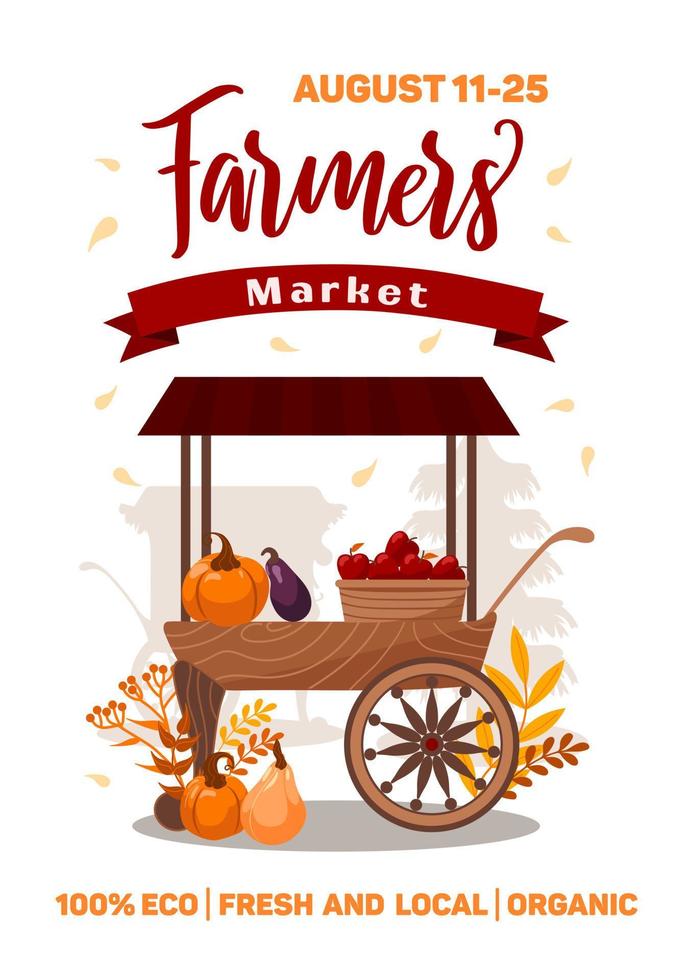This image is an advertisement poster for a farmer's market running from August 11th to 25th. At the top, in bold orange capital letters, it announces the date range. Below the dates, the word "Farmers" is written in a dark reddish script font with a capital "F." Underneath "Farmers," the word "Market" is displayed on a crimson red banner in white capital letters. The focal point of the poster is a stylized, vector-like illustration of a pushable food cart featuring a large central wheel. The cart is laden with fresh produce, including a pumpkin, an eggplant, and a basket of red apples. Additional pumpkins, squashes, and yellow and orange autumn foliage adorn the ground around the cart. The background features scattered beige-yellow leaves, enhancing the fall theme. At the bottom, the poster declares the produce to be "100% eco, fresh and local, and organic" in bright orange font. The overall color scheme is dominated by warm, fall-inspired tones of orange, brown, and red, giving it a vibrant, seasonal feel.